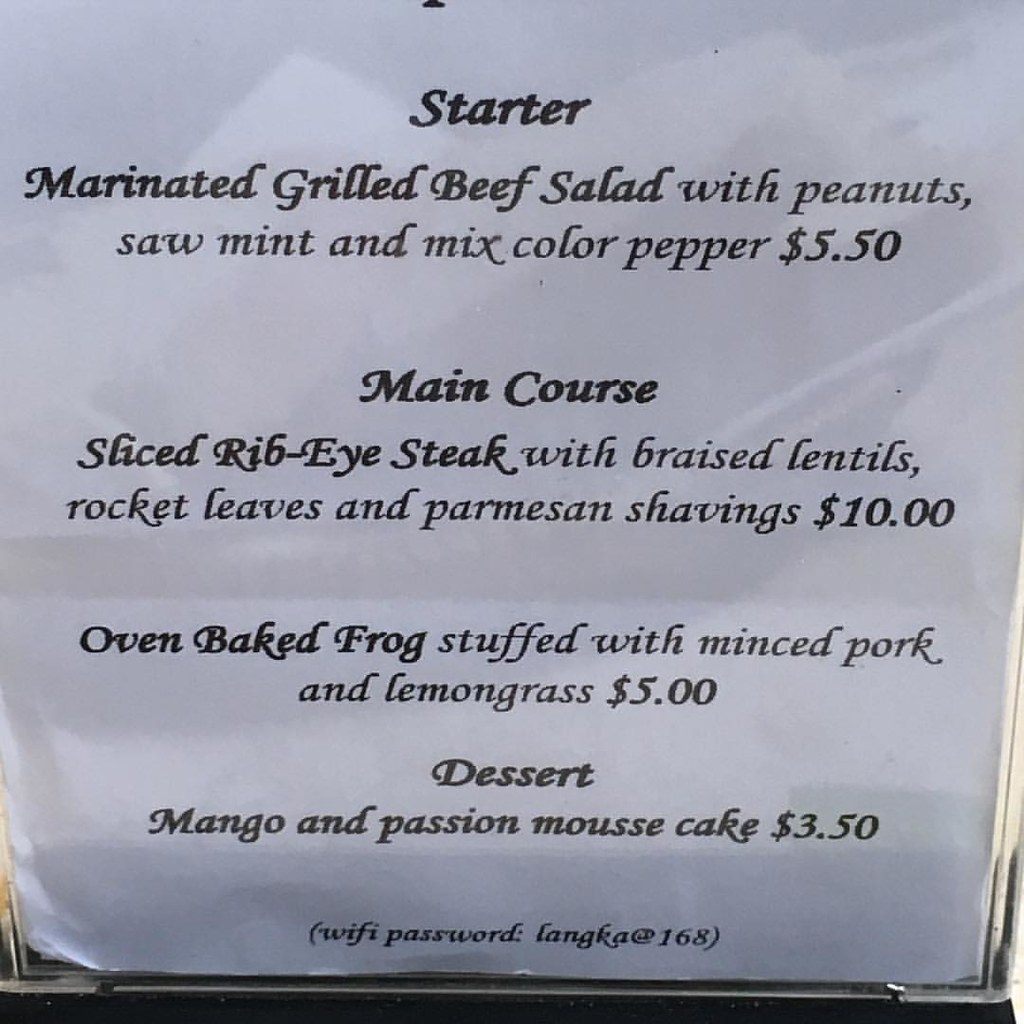The image depicts a simple yet detailed menu encased in plastic. At the very top, the menu lists its categories starting with "Starter." The first item is a "Marinated Grilled Beef Salad" featuring peanuts, mint, and mixed colored peppers, priced at $5.50. The "Main Course" section follows with "Sliced Rib Eye Steak with Braised Lentils, Broccoli, and Provolone Shavings" for $10, and "Baked Frog Stuffed with Minced Pork and Lemongrass" at $5. The "Dessert" section offers a "Mango and Passion Fruit Steak" for $3.50.

The bottom of the menu, in parentheses, includes the Wi-Fi password: "LAGKA168." The menu is printed on white paper with cursive text, some parts bolded and others not. It seems to have been through some wear, highlighted by the noted trading issues on the paper and the condition of the corners, particularly the bottom left. The whole menu is encased in plastic, suggesting it is part of a display, possibly not meant to be handled directly but rather viewed from within its protective encasing. This simple menu does not feature many items, but it provides clear and concise information.